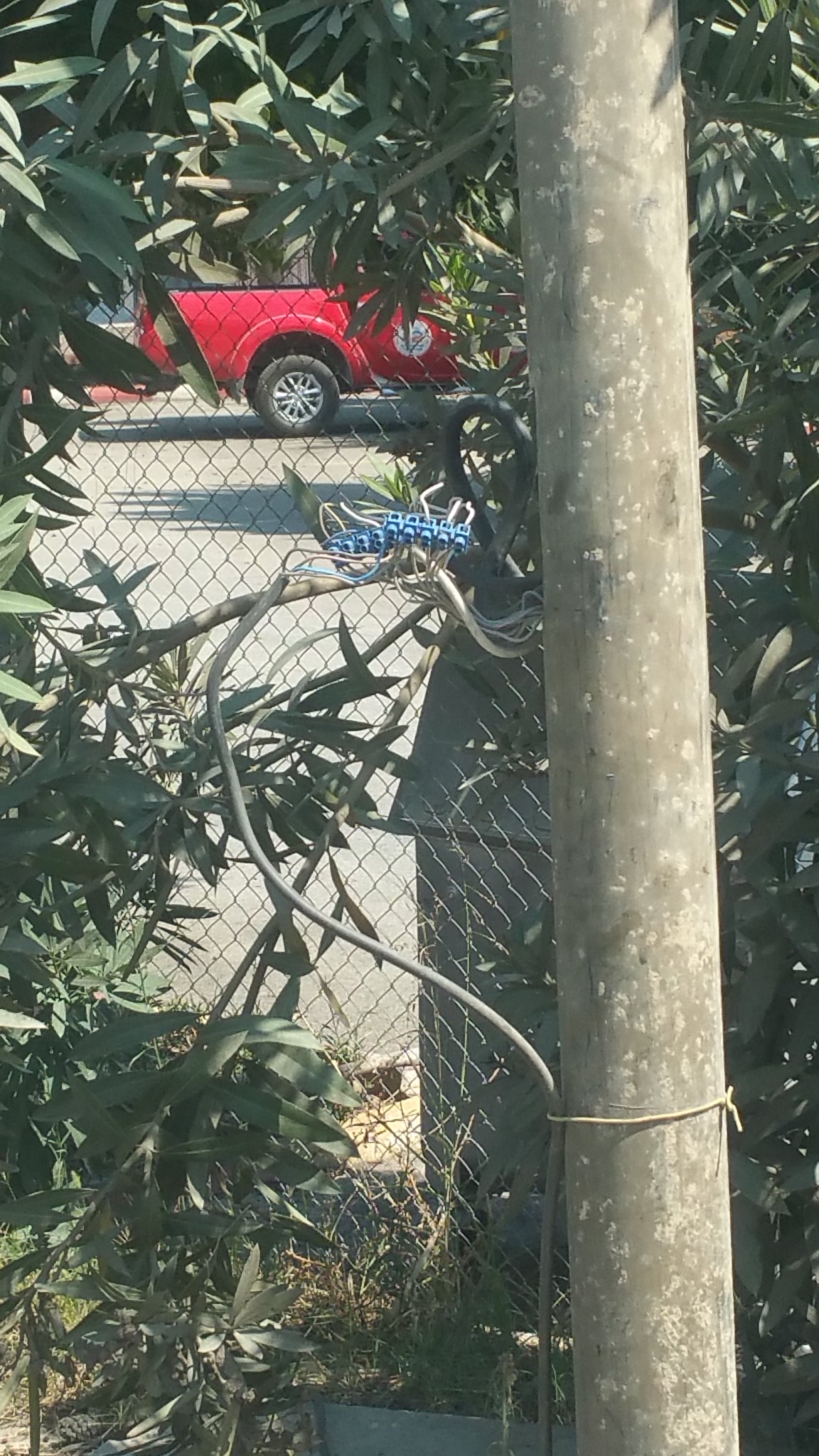The photograph, in color and portrait mode, captures a scene through a chain link fence situated in what appears to be a yard. Dominating the left side of the image is a metal utility pole, around whose base is a string supporting a plant, guiding its upward growth. This plant appears as just a branch amidst the surrounding green foliage. The unkept grass at the bottom and various plants create a natural frame around the central elements. In the background, beyond the metal chain fence, a red pickup truck is partially visible, showing only its back end and a wheel with an indistinct logo. Adjacent to the pole, there is a hint of blue plastic connected to electrical wiring, and a trash can can be seen nearby. Further back, a stretch of pavement is seen, suggesting a road or driveway beyond the yard.